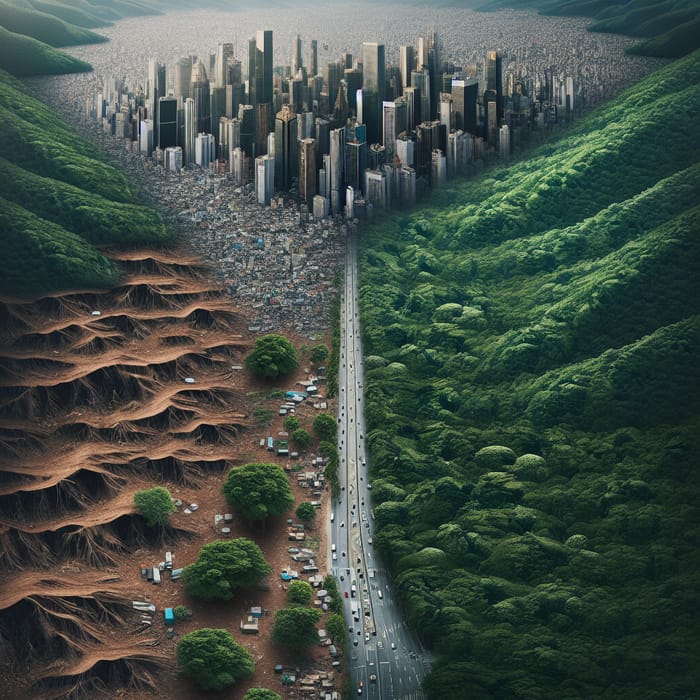In this AI-generated digital art piece, we see a sprawling, urban landscape from a bird's-eye view. The image is rectangular and centered around a multi-lane highway that stretches from the bottom center and travels upwards, cutting through diverse terrain before reaching a dense cityscape in the top 20% of the frame. The city is characterized by towering skyscrapers centralized in a diamond-like formation, surrounded by smaller suburban homes and slum-like structures that extend into a vast valley.

On the left side of the image, the terrain is barren and rugged, featuring multiple dirt levels with sparse vegetation, such as scattered trees and shrubs mostly concentrated at the base and upper sections. Numerous parked cars are visible alongside the road on this bare, earthen expanse. In contrast, the right side is lush and fully green, dominated by thick vegetation that covers the mountainous area.

The city itself is set within this green valley, with the central high-rise buildings giving way to smaller structures as one moves outward. The surrounding suburbs fade into indistinct hills and gullies, covered with grass and trees. Numerous cars populate the highway leading into the city, emphasizing the bustling activity of this metropolitan hub.